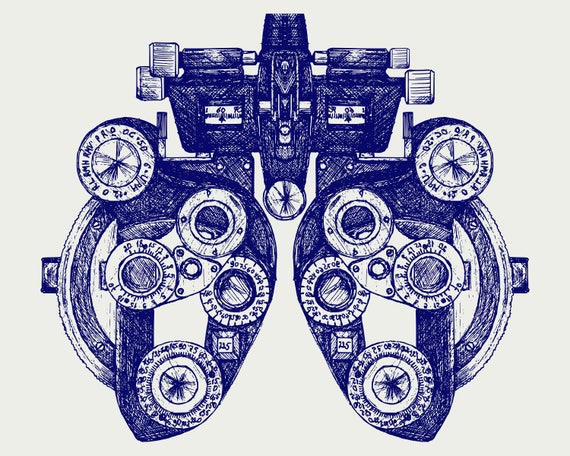The image depicts a detailed blue-on-white drawing of an optometrist's phoropter, an instrument used for testing eyesight. The drawing is rendered in blue ink on a white background, with light and dark blue shades providing depth and contrast. The phoropter features two main circular sections on the left and the right, each filled with numerous numbered lenses and dials. These sections are connected by an upper segment that also houses additional dials, resembling a bridge. The instrument, which looks somewhat like goggles with a series of different circular lenses attached, has a symmetric design, with identical left and right parts. The intricate arrangement of lenses and dials gives it the appearance of a streamlined object, somewhat akin to the front of a sports car, with "tires" on either side in the form of large, turning dials and a central streamlined body.